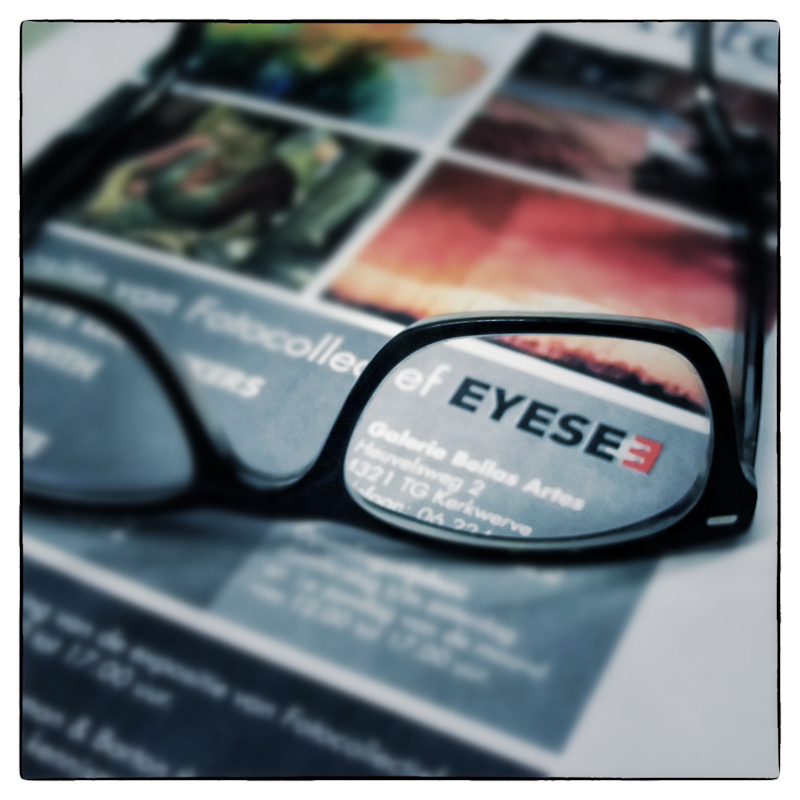The image showcases a close-up photograph possibly meant for an advertisement, displaying a pair of black plastic-framed eyeglasses positioned upside down on a white pamphlet or magazine, likely lying on a table. Through the lenses of the glasses, the text "EYESE" followed by a backwards "E" can be seen, where all letters are black except the red backwards "E." The pamphlet features four rectangular photos, one of which depicts a sunset skyline, while the others are not clearly identifiable. Additionally, the pamphlet bears a gray box containing more text, which seems to include details such as "IC" and a possibly associated address, "1321 TG Kirkworth," though some of the text is blurred and difficult to decipher.